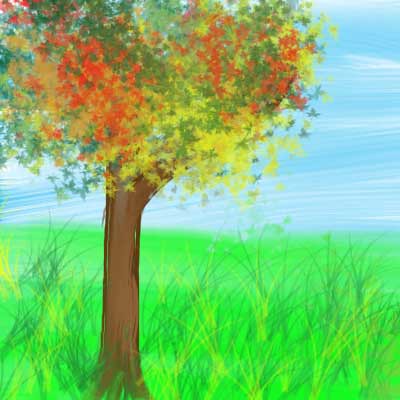This watercolor painting depicts a tranquil outdoor scene on a sunny day. The sky is rendered in soft blue tones, with white brushstroke clouds leisurely drifting across. Lush green grass covers the lower half of the composition, with long, crisscrossing blades appearing to sway gently in a mild breeze. Toward the right-hand side, a tree stands gracefully, its trunk and a prominent branch extending leftwards. The tree's foliage is a delightful mix of autumnal hues — rich reds, vibrant yellows, warm oranges, and lingering greens. Amidst the greenery, subtle touches of yellow add to the depth and variation of the grass. The artist's skillful use of watercolor imbues the scene with a sense of peace and gentle movement, perfectly capturing a serene moment in nature.